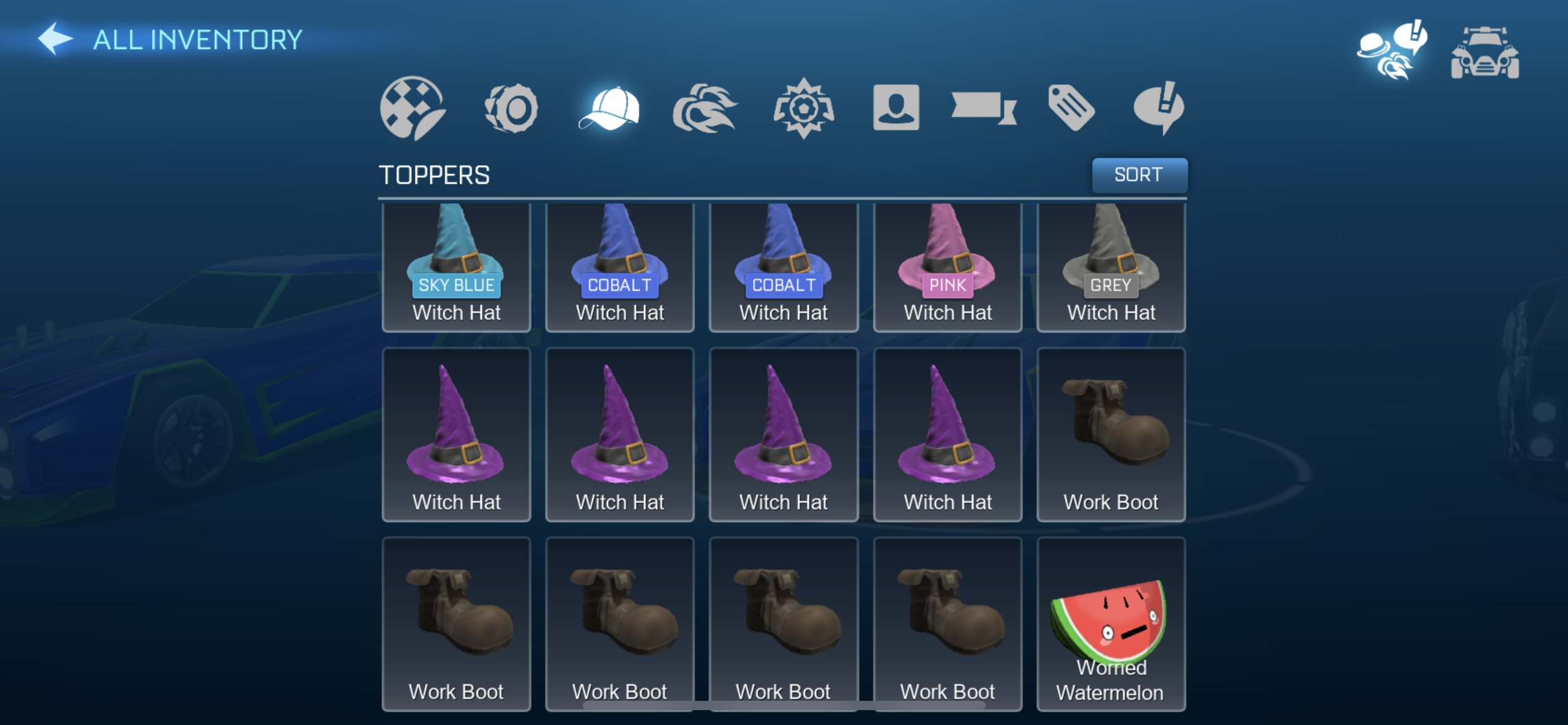The image appears to be a screenshot from a video game interface, featuring a teal background with a faint car outline, possibly in purple or royal blue with yellow accents. 

In the top left corner, the glowing text "All Inventory" is accompanied by a white arrow. The upper right corner of the screen displays several icons, including a car, a top hat, a speech bubble with an exclamation mark, and other miscellaneous icons.

An icon-type menu spans the top middle of the screen, showcasing various avatar-like images: a round checkerboard, a tire, a ball cap (highlighted brightly), flames, a user icon (a silhouette of a person), a sideways banner/ribbon, a luggage or price tag, and a speech bubble with an exclamation mark.

Below this menu, the section titled "Toppers" is followed by a "Sort" tab on the right side. The main display area shows three rows of items: 

1. The first row features witch's hats in various colors such as sky blue, cobalt, pink, and gray, totaling five hats with two appearing cobalt.
2. The second row continues with more witch's hats in colors like purple and an additional work boot.
3. The third row displays four work boots of different colors and a slice of watermelon with eyes, mouth, and an anxious expression.

These items, arranged for selection, suggest customizable options possibly used within the game environment, hinting at a fantasy or VR context.